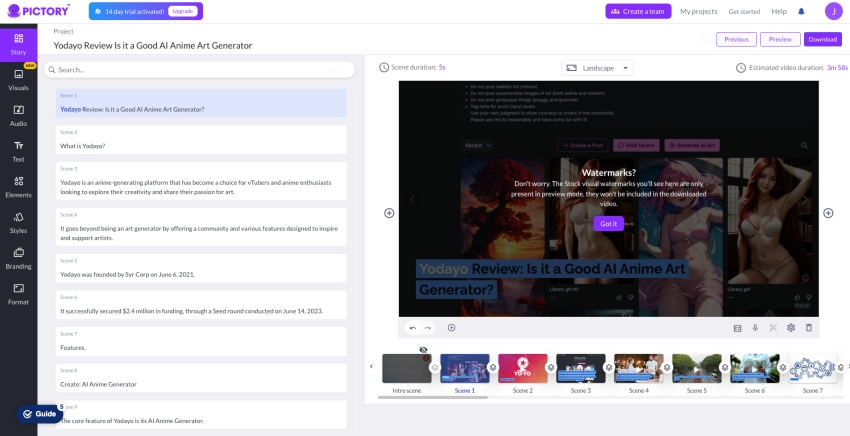The image depicts a user interface with a white background. At the top center, the word "Pictory" is displayed in purple, accompanied by a small purple icon featuring a circle with a block underneath. Below this, a blue search box is prominently positioned.

On the right side of the interface, there's a purple button labeled "Create," followed by the options "My Projects," "Get Started," and "Help." Adjacent to these, icons of a blue bell and a purple clock are visible. Further down on the right side, there are three additional buttons: two white with purple text, and the last one in purple.

On the left side, a long black box extends downward, with a purple box labeled "Story" at the top. A small yellow tag marked "New" is attached to this section. Alongside the left edge, there are six or seven small icons. At the bottom of this black box, a blue button labeled "Guide" is present. To the right of this button, the text "Yodeo Review: Is it a good AI anime art generator?" is displayed next to a search button.

Below this area, the interface includes a light blue box containing a sentence, followed by a white box and seven more white boxes with text in them. On the right side, there's a section for "Scene Duration" with a clock icon, a "Landscape" dropdown menu, and another clock icon.

A significant feature in the center is a large picture with a dark background. It shows a central circle with a plus sign on either side, surrounded by four smaller images with white watermarks. Beneath this, a purple "Got it" button and blue text stating "Yodeo Review: Is it a good AI anime art generator?" are visible. Finally, a light blue button with various small icons, a white box with eight smaller boxes containing different pictures complete the interface elements.